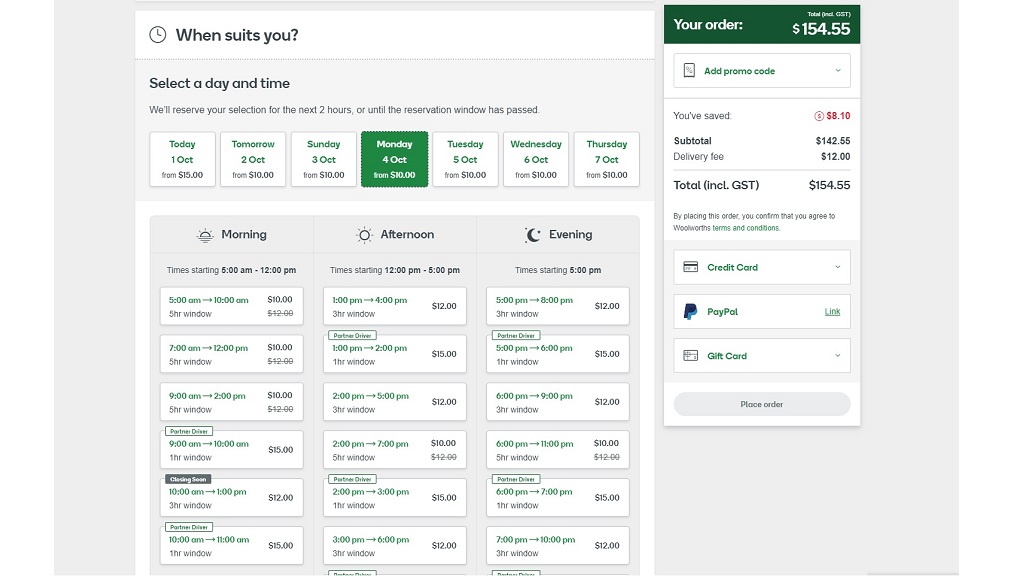The image depicts a complex user interface split into two distinct sections. The left side features a calendar or agenda planner with a search bar at the top containing the query "when suits you." Users can select a specific day and time, as illustrated by the date Monday, October 4th, with available options starting from $10. This section seems to offer various scheduling possibilities, likely related to booking travel services such as flights or hotel stays. On the right side of the image, there is a checkout area indicating the order total of $154.55, a promo code field, a savings display of $8.10, and options for selecting a payment method and placing the order. This detailed layout suggests a comprehensive booking system that integrates scheduling and payment functionalities seamlessly.